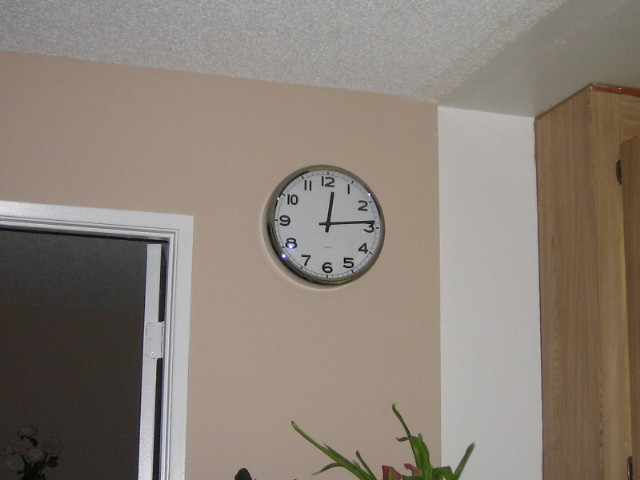The image depicts an indoor scene focused on a wall clock. The clock, displaying the time 12:14, has a white face with black numbers and hands, and is encased in a shiny silver frame. The clock is mounted on a light tan, almost peachy, wall which transitions into a white wall, dividing two different rooms. To the right of the clock, a tall wooden cabinet extends up to the ceiling, made from light brown wood. In the bottom left corner of the image, there's a doorway; however, it is too shadowed to discern the contents within that room. Framing the lower edge of the photo, the green stems and occasionally visible pink flowers of a plant add a touch of nature to the indoor setting. The overall image blends domestic details harmoniously, emphasizing the central clock against its backdrop.